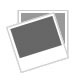This is a detailed, close-up photograph of two folded blankets, likely woven from thick yarn or thread. The blankets, stacked one on top of the other, feature a plaid-like pattern composed of earth tones, including shades of dark brown, light brown, orangey-brown, reddish-orange, and tan. One corner of the top blanket is folded over towards the viewer, revealing fringes that match the blanket's color scheme. The fringes, approximately four inches long, hang freely from the edge. The blankets are set against a stark, featureless white background that emphasizes their intricate cross-stitching pattern; the horizontal stitching is lighter, while the vertical stitching is in darker earth tones. The photo captures the texture and woven details of the blankets, identifying them as modern and without any wording or symbols.